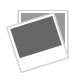This image showcases a vintage marketing pin set against a textured gray and white woven background. The pin is oval in shape with a pale lemon yellow background and features an intricate border in pale gold. It appears to be well-worn, exhibiting several nicks and areas where the paint has chipped off. Central to the design is a split image of a rocket, the top tip of which angles toward the lower right of the image. The rocket, detailed in black with dark gold edging, is broken in two segments by the letters "H-E-T," which are arranged diagonally from the lower left to the upper right in a pale blue color, also outlined in dark gold. There's an "N" on the nose of the rocket. The rocket's bottom segment appears implanted in the oval, evoking a sense of the pin resembling a planet. The combination of these elements—gold detailing, pale blue lettering, and the split rocket design—creates a compelling, albeit aged, piece of memorabilia.